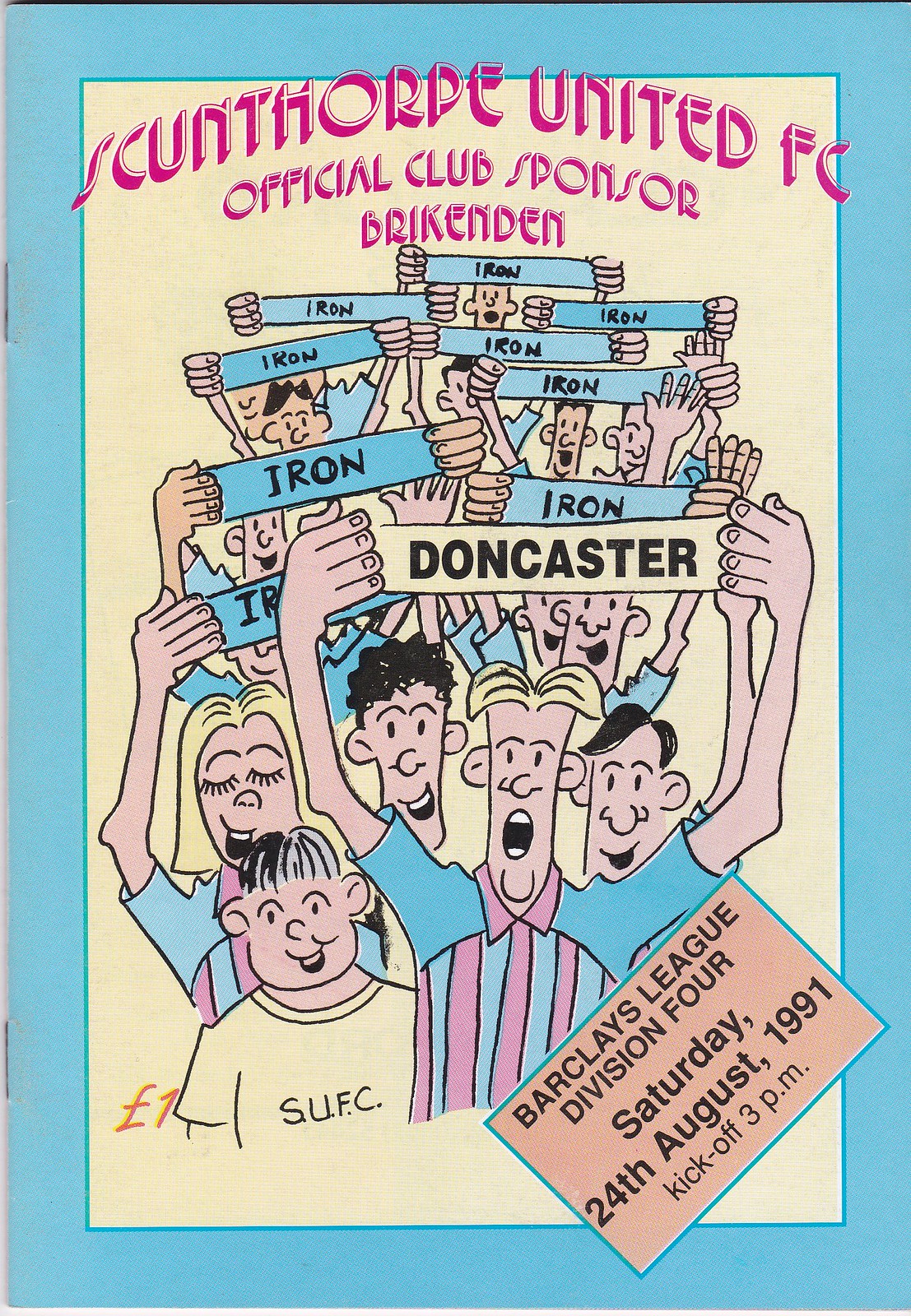The image is a tall rectangular front page of a sports program, bordered by a light blue outline with staples at the top and bottom on the left edge. The inner section features a light yellow background with curved magenta text at the top reading "Scunthorpe United FC Official Club Sponsor Brickenden." Below, a cartoon illustration depicts several rows of people, mostly fans, holding up signs. Their shirts alternate between yellow and pink-and-blue stripes. The majority of the signs are blue with the word "Iron," except for one prominent yellow sign in the front which reads "Doncaster." To the right of the person holding the yellow sign, another character in the crowd wears a shirt that says "SUFC" and has distinctive stringy hair. Also included is a pinkish rectangle at the bottom right, indicating "Barclays League Division Four, Saturday 24th August 1991, Kickoff 3 p.m." The overall look of the program, with its faded colors and dated design, suggests it is an old soccer match booklet from the 1990s.